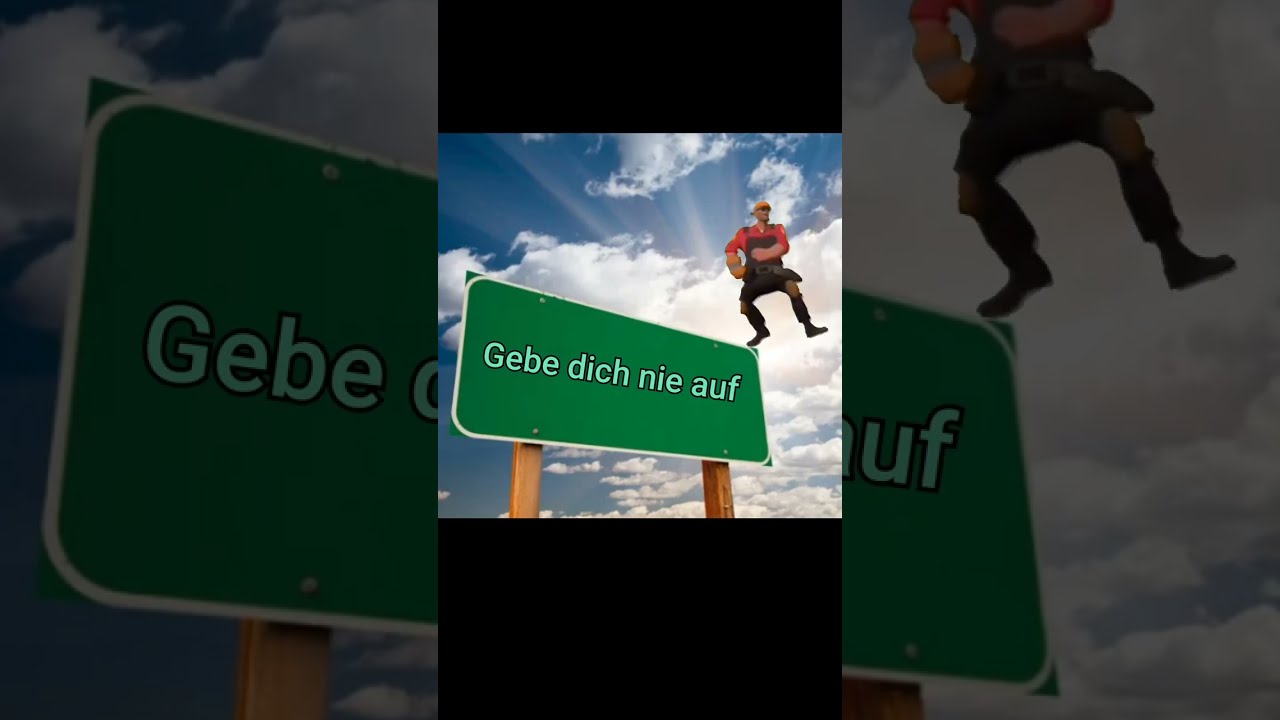In this image, there's a 3D-rendered video game character resembling a construction worker or a Mario-like figure, wearing a red shirt, dark overalls, a hard hat, brown pants, and boots. He stands prominently in the upper right portion of the image, seemingly balanced on the edge of a green street sign held aloft by wooden posts. The sign, outlined in white, contains German text which reads "Gib dich nie auf" (translated as "Never give up"). The background depicts a vibrant sky with rays of sunlight piercing through white clouds, adding a heavenly aura to the scene. The image itself is framed by thick black bars at the top and bottom, giving it the appearance of a meme or an advertisement.